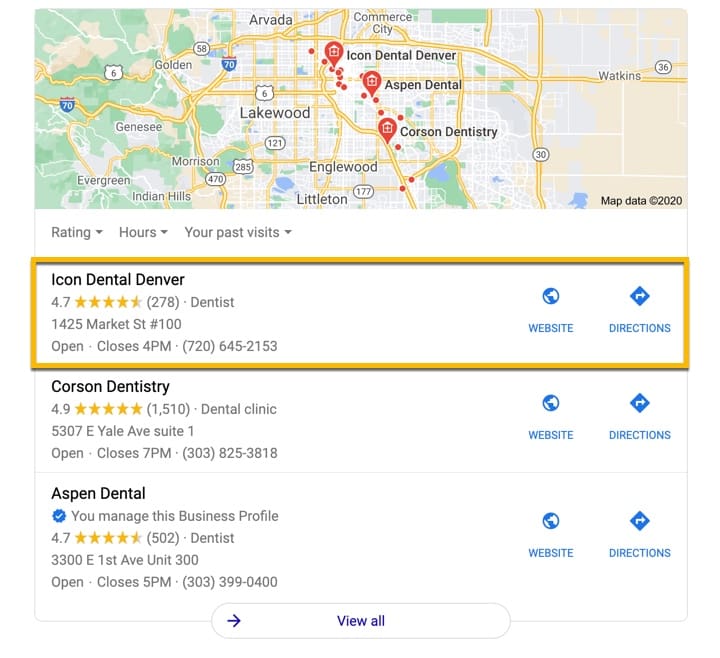This Google Maps screenshot displays dental care providers in Colorado, highlighting three prominent locations: Icon Dental Denver, Aspen Dental, and Corson Dentistry. The map is dotted with a total of 20 location markers representing various dental practices.

The highlighted dentists are further detailed in individual listings below the map. Icon Dental Denver, rated 4.7 out of 5 based on 278 reviews, offers links to its website and directions. Corson Dentistry boasts a high rating of 4.9 stars from 1,510 reviews and also provides website and directions links. Aspen Dental, verified with a blue checkmark, has a 4.7-star rating from 502 reviews, accompanied by links to its website and directions.

A "View All" button is available for users who wish to explore additional dental profiles.